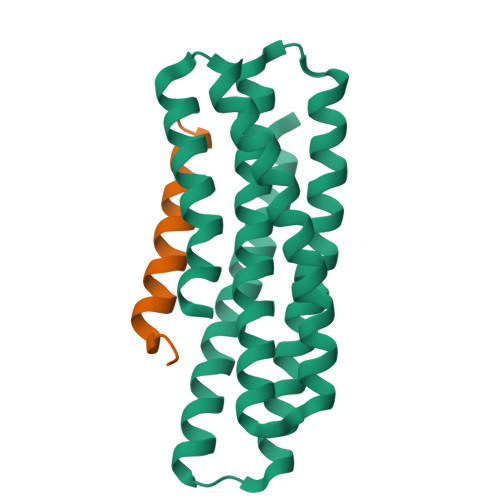The photograph showcases vertical spiraling ribbons against a stark white background. On the left side, there is an orange ribbon, while the right side features five green ribbons, each twirling in a corkscrew pattern. These ribbons vary in length, with some being longer and others shorter, with one green ribbon being the same length as the orange one. The tops of all the ribbons are connected, and some are also joined at their bottom ends, possibly with a thread or wire. The spirals are distinct, lending a dynamic and playful look to the image.